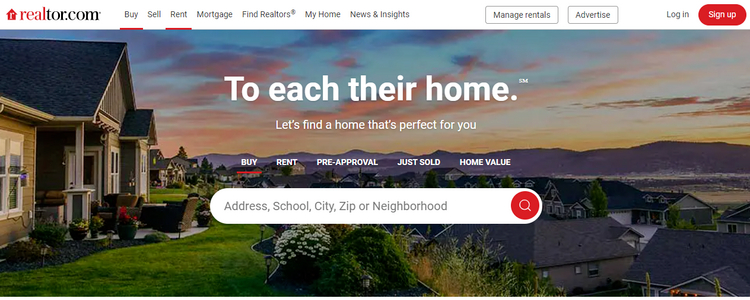A picturesque residential hillscape in Edmonton showcases a charming row of houses with gray rooftops nestled amid lush greenery. The foreground features vibrant green lawns adorned with white flowers and inviting sitting areas, perfect for enjoying the scenic views. Background visibility includes majestic mountains and a clear blue sky, sporadically decorated with clouds. This image invites you to explore and find your dream home, highlighting the ideal setting for buying, renting, or obtaining mortgage pre-approval through realtor.com.